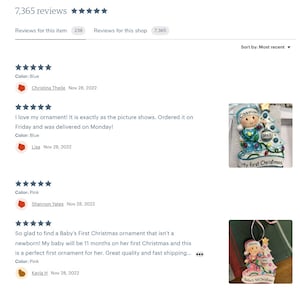The image depicts a webpage with a white background that highlights product reviews. At the top, it prominently displays "7,365 reviews" accompanied by five black-shaded stars, indicating a high rating. Below the stars, there are two headings: "Reviews for this item" and "Reviews for this shop." 

On the right side of the page, there's a section for sorting reviews, labeled "Sort by: Most Recent," with a dropdown arrow beneath it. The reviews are listed below:

1. The first review shows five stars and mentions "Color: Blue."
2. The second review, also with five stars, reads: "I love my ornament. It is exactly as the picture shows. Ordered it on Friday. It was delivered on Monday. Color: Blue."
3. Another five-star review simply states "Color: Pink."
4. The final review, rated five stars, says: "So glad to find a baby's first Christmas ornament that isn't a newborn. My baby will be 11 months on her first Christmas. This is a perfect first ornament for her. Great quality and fast shipping."

Note: Some text on the page appears blurred and difficult to read, making certain details unclear.